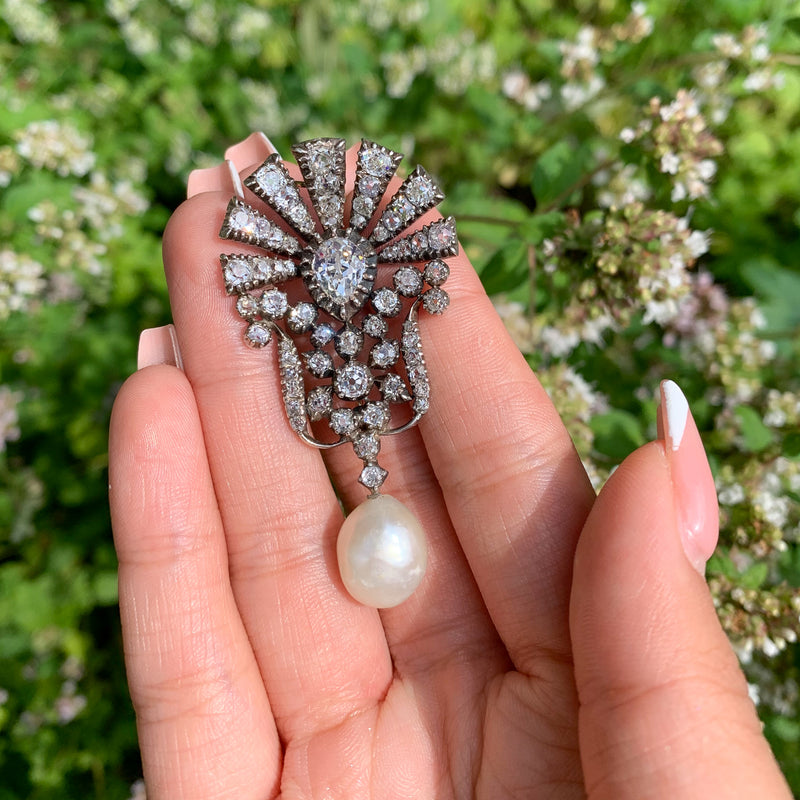In this photograph, we see a well-manicured hand, likely a woman's, adorned with long, pink fingernails featuring white tips—a classic French manicure. The hand is holding an ornate brooch, prominently showcasing a large central diamond. Radiating from this central diamond are bars of smaller, sparkling diamonds, giving the appearance of rays around a setting sun. Underneath these radiant bars are circular arrangements of additional diamonds. At the very bottom of the brooch, a single, elegant white pearl dangles. This hand, showing visible wrinkles and positioned palm-up, extends from the bottom of the image toward the upper left. In the background, there are indistinct, green leafy plants adorned with sprigs of white and purplish flowers, adding a natural touch to the intricately held piece of jewelry.